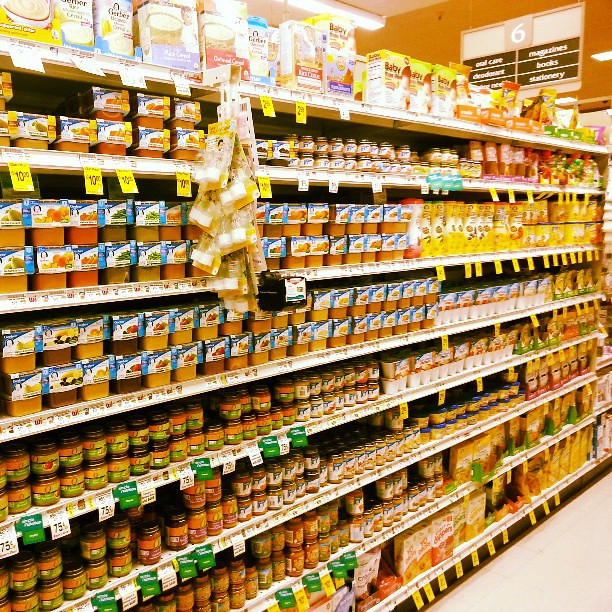This image is a color photograph taken inside a supermarket, depicting the perspective of an aisle. The scene captures a row of multiple shelves arranged diagonally from the left front toward the right back of the frame. A sign is visible hanging from the ceiling in the top right corner of the image, sporting a large white number 6. The sign lists six different items to help shoppers locate specific products in the aisles: oral care, magazines, books, and stationery are readable despite being slightly blurred.

The aisle in focus appears to be either aisle 5 or 7, primarily stocked with food items. The shelves are nearly completely full, prominently featuring jarred food products, including baby food and possibly salsa, recognizable by some branding logos such as Gerber. Various containers, likely of food items, occupy the second shelf from the top downwards, with medium-sized jars lining several subsequent shelves. The bottom shelf holds packets or boxes of other food items, with yellow labels hanging down from plastic strips on the edge of each shelf, indicating prices or discounts. The ceiling above shows a long fluorescent light fixture, adding to the supermarket ambiance.